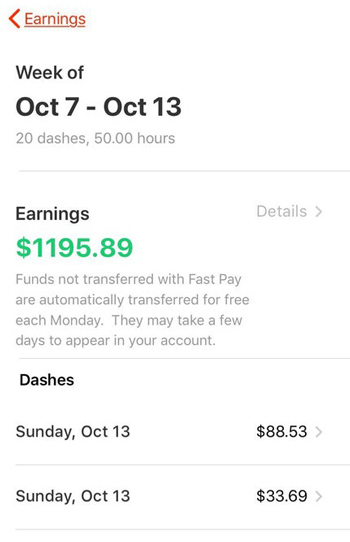The image displays a webpage titled "Earnings" with a back button located near the top. The period covered is from October 7th to October 13th, and it documents 50 hours of work, presumably for DoorDash. The total earnings for this period amount to $1,195.89. It includes a note indicating that funds not transferred using FastPay are automatically transferred for free each Monday, with a processing time of a few days before appearing in the account.

A detailed breakdown for each day or each order is listed below. Notably, on Sunday, October 13th, there are two entries showing earnings of $88.53 and $33.69, respectively. These figures likely represent the daily earnings, indicating a substantial amount of income generated. Over fifty hours, the earnings seem significant, allowing for a sustainable living assuming a reasonable cost of living.

The webpage is designed with a white background and black font, except for the total earnings figure which is highlighted in green for emphasis.